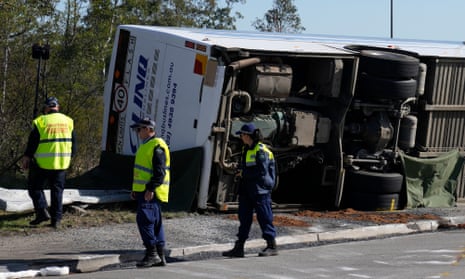The image depicts an overturned bus lying on its side on a sidewalk adjacent to the road, partly resting on some grass. The bus, primarily white, shows the number 40 at the top of its back end and has some writing visible. The back four wheels are prominently displayed. The scene is set against a backdrop of trees visible to the left. In the foreground, a concrete curb and sidewalk can be seen. Three workers are present, all dressed in blue pants, black boots, and reflective yellow vests with silver stripes. Their upper attire includes blue long-sleeved shirts and hats. Two of the workers appear to be men, while the third is a woman. The workers are positioned near the upturned vehicle, seemingly assessing the situation.